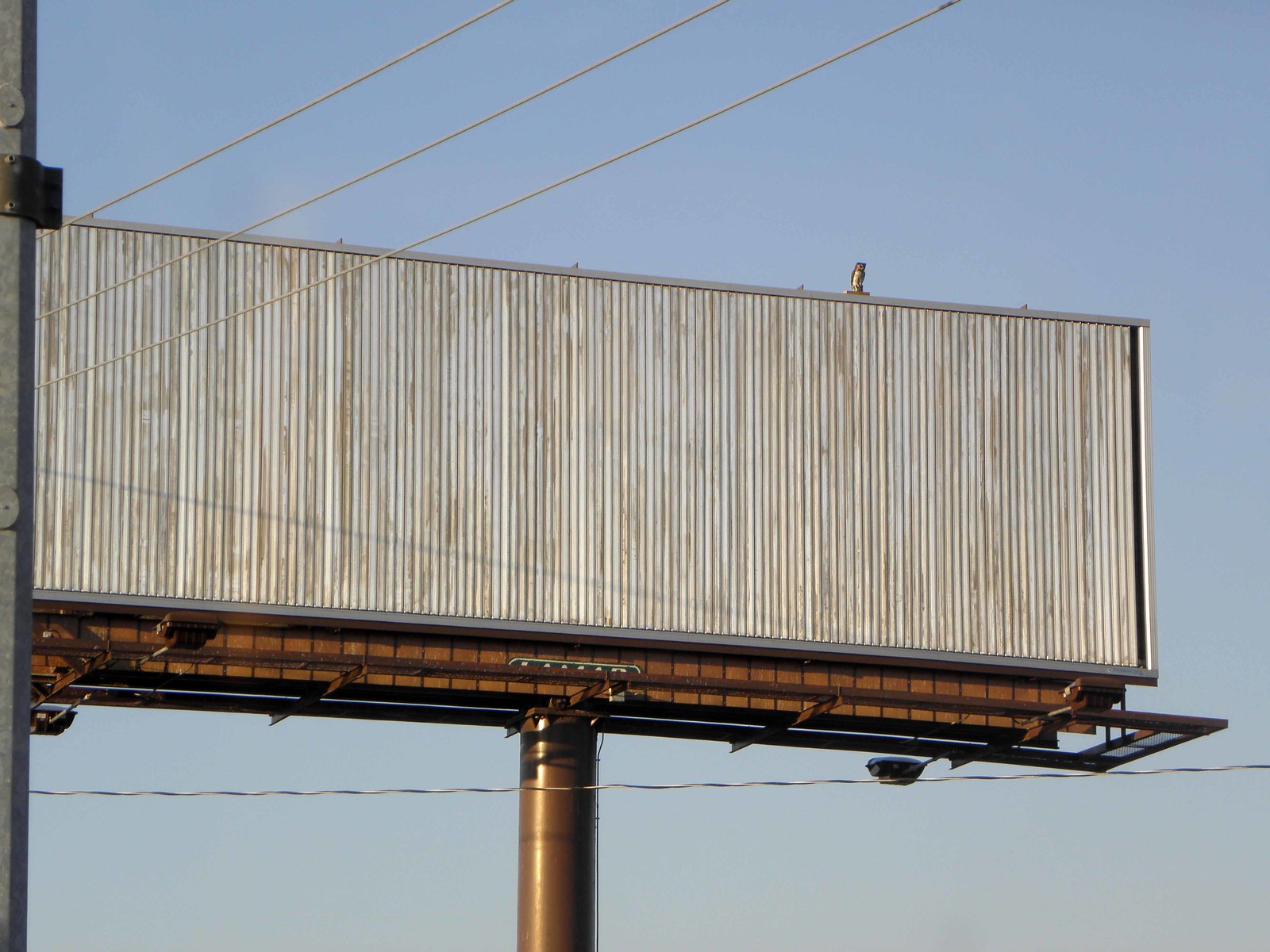A towering highway billboard stands elevated on a circular support, lifting it high into the air. The billboard boasts a large display area designed for rotating vertical strips, allowing it to cycle through three or four different messages periodically. Below the display, there is a platform where workers can safely stand to change the ad content. Overhead, power lines intersect the image, running from the top to the mid-left edge, while a lone telephone wire stretches horizontally near the bottom. Against the backdrop of this bustling highway advertisement, a clear, cloudless blue sky extends infinitely, providing a serene contrast to the industrial elements in the foreground.